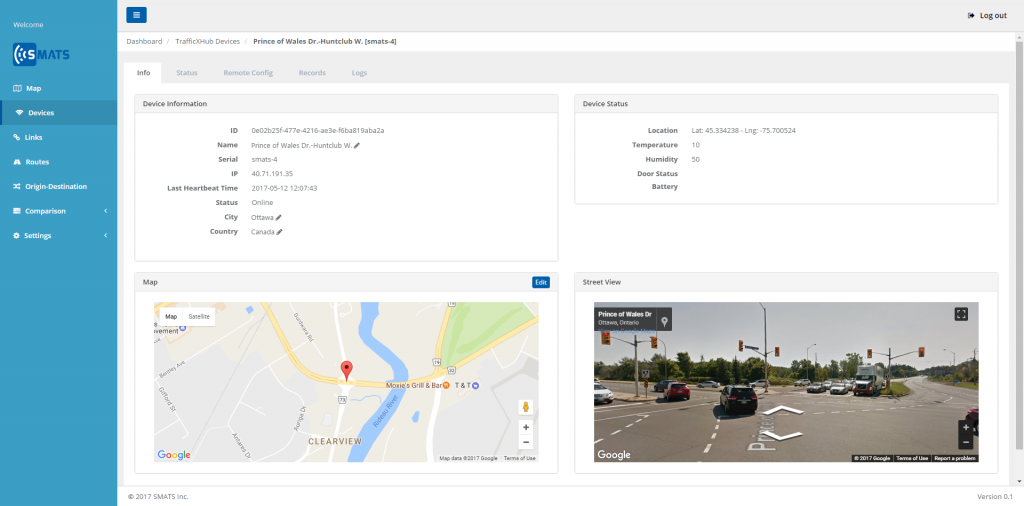The image depicts the interface of a website named SMATS. The left side features a blue vertical sidebar with a collection of headings, albeit in small font, which makes them somewhat difficult to read. These headings include options such as "Map", "Original Destination", "Comparison Settings", and "Links". The current selection in the menu appears to be "Devices".

On the right side of the interface is a main panel dominated by a white background with grey sections containing various headings. This section provides detailed information about devices, broken down into categories like "Device Information" and "Device Status". Specific attributes listed under "Device Information" include location, temperature, humidity, driver status, battery level, name, serial number, and city.

Beneath this information, a zoomable map resembling a standard Google Map is displayed. Adjacent to the map on the right is a street view representation, offering a more detailed and immersive view of the map area. The design and layout provide a comprehensive overview of device data alongside geographic and street-level mapping features.